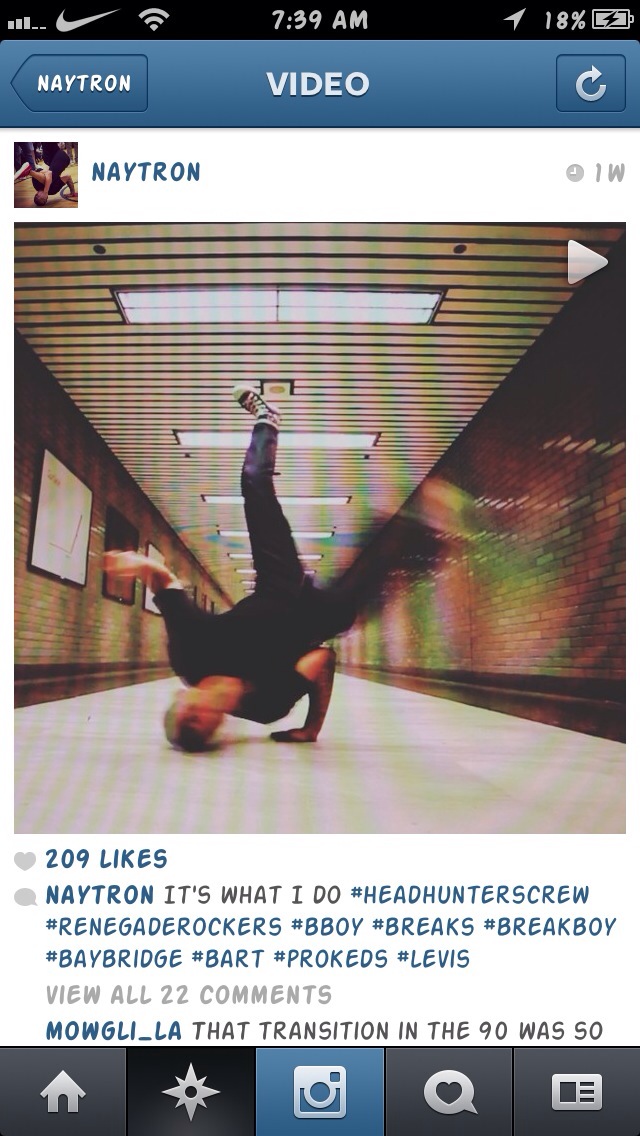This is a detailed screenshot of a social media app on a smartphone, showcasing a video of a person breakdancing in a narrow, brick-lined hallway adorned with framed images on the left side. The breakdancer, wearing a black short-sleeved shirt, dark blue jeans, and black and white Converse sneakers, is captured mid-move with his head down and legs up in the air. At the top of the screen, a small blue band reads "Video," with "Navtron" on the left and a refresh button on the right. Above this, the smartphone's status icons are visible, including the time, active signal strength, battery percentage, and a Nike logo. Beneath the video, the screen shows 209 likes, followed by hashtags such as #Headhunters Crew, #Renegade Rockers, #B-Boy, #Breaks, #Break Boy, #Bay Bridge, #Bart, #Pro-Kids, and #Levi’s. There's a prompt to "View all 22 comments," with a visible comment that starts with "Mowgli_underscore_LA: that transition then in the 90s was so…" but is cut off. At the bottom of the screen, standard navigation buttons are also visible.